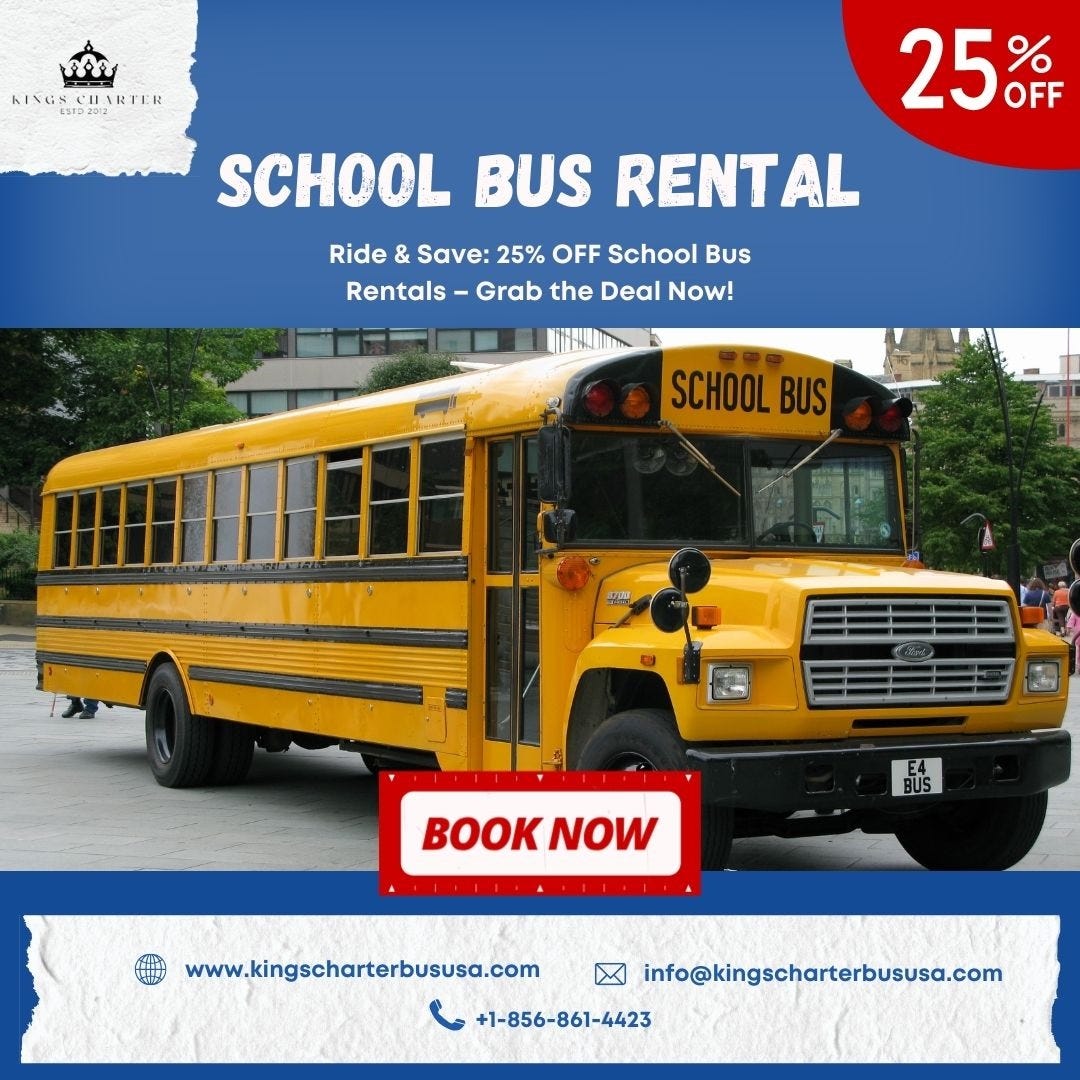This advertisement for King's Charter school bus rental prominently features a bold design. At the top left corner, a red quarter-circle background with white text announces "25% off." Adjacent to this, "King's Charter" is written along with a small crown symbol. The central part of the advertisement has a blue background with white text stating "School Bus Rental." Below this, it reads "Ride and save 25% off school bus rentals. Grab the deal now." Positioned beneath the text is an angled photograph of a classic yellow school bus, showcasing both its length and front. Situated below the front right wheel of the bus is a "Book Now" prompt in red on a white rectangle. The bottom portion of the ad includes another blue stripe with white details, providing the website www.kingscharterbususa.com, the email address info@kingscharterbususa.com, and the phone number +1-856-861-4423, all written in blue text on a white background.